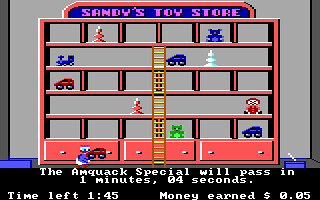This image depicts a retro-style arcade or video game screen. The main focus is a vibrant, red shelving unit with multiple levels. At the very top of the shelf, a sign reads "Sandy's Toy Store" in bright pink letters, adding a whimsical touch. A central ladder extends upward, flanked by red drawers at the base of the shelving.

Perched on the bottom shelf is a character resembling Donald Duck, who is holding a red toy car. Below this charming scene, white text informs the player that "The AmQuack special will pass in one minute and four seconds," suggesting a timed event or challenge within the game.

Additionally, two indicators are displayed on either side of the screen's lower part. On the bottom left, a time indicator shows "Time left: 1:45," counting down the remaining gameplay duration. On the bottom right, it states "Money earned: $0.05," tracking the in-game earnings. This nostalgic scene captures the essence of classic arcade gaming with its playful design and engaging details.